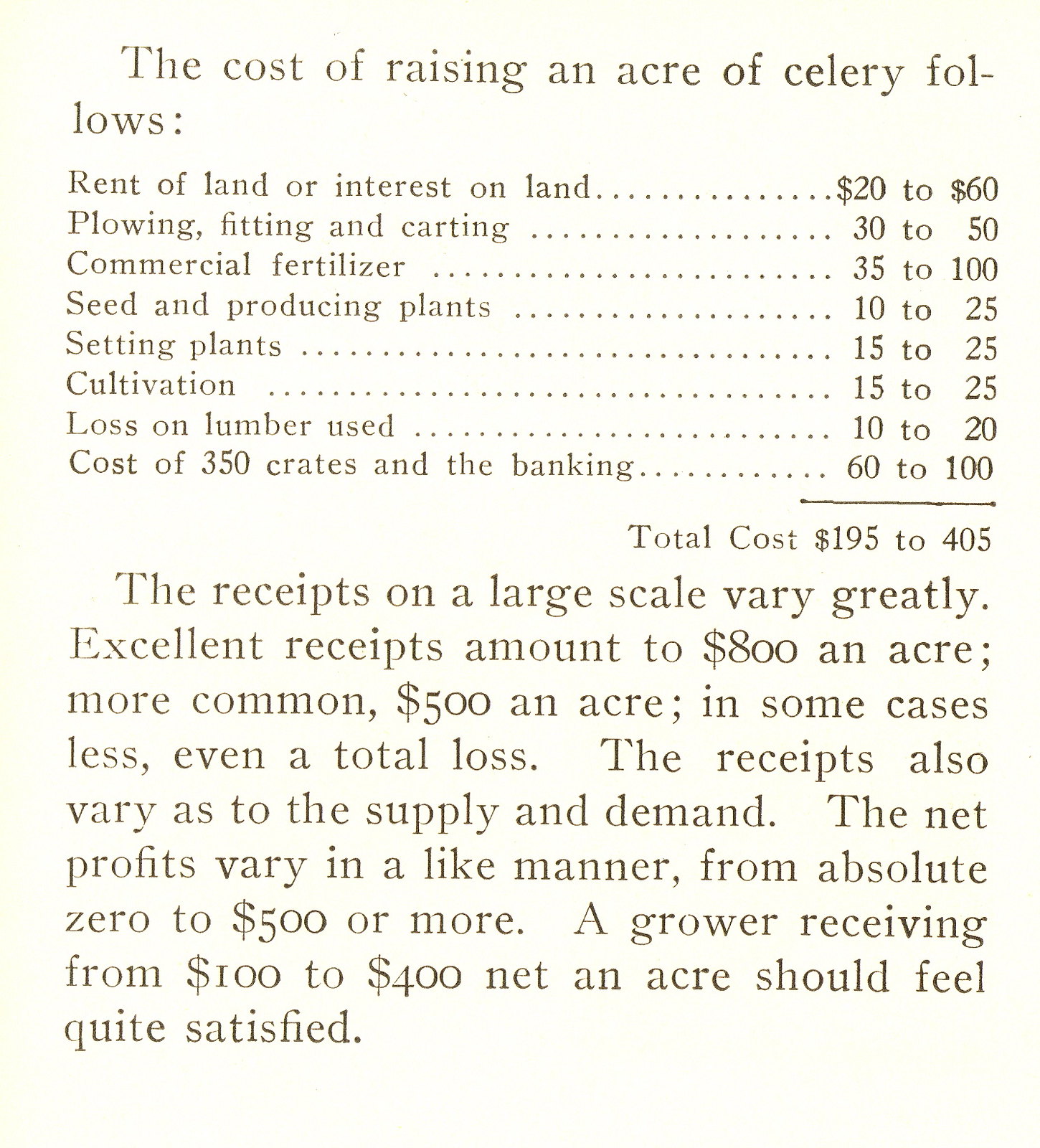The image depicts an old, weathered document, possibly from a book or magazine, with a headline that reads in large, bold text: "The Cost of Raising an Acre of Celery." The background is a very pale, tan-colored paper. Below the heading, in smaller text, the document systematically lists the various expenses involved:

1. Rent of land or interest on land ........ $20 to $60
2. Plowing, fitting, and carting ............... $30 to $50
3. Commercial fertilizer .......................... $35 to $100
4. Seed and producing plants ................. $10 to $25
5. Setting plants ...................................... $15 to $25
6. Cultivation............................................. $15 to $25
7. Loss on lumber used ........................... $10 to $20
8. Cost of 350 crates and banking .......... $60 to $100

Total cost ranges from $195 to $405.

The passage further details the potential receipts from raising an acre of celery, highlighting that returns vary significantly. Excellent receipts can reach $800 per acre, while more common returns are around $500 per acre. However, it's noted that in some cases, the returns could be so poor that they result in a total loss. The net profit is influenced by supply and demand and can range from nothing to $500 or more per acre, suggesting that a successful grower could expect a net profit between $100 to $400 per acre and should feel quite satisfied with these figures.

This detailed breakdown is presented in black text on a white to tan background, lending the document an antique and informative appearance.